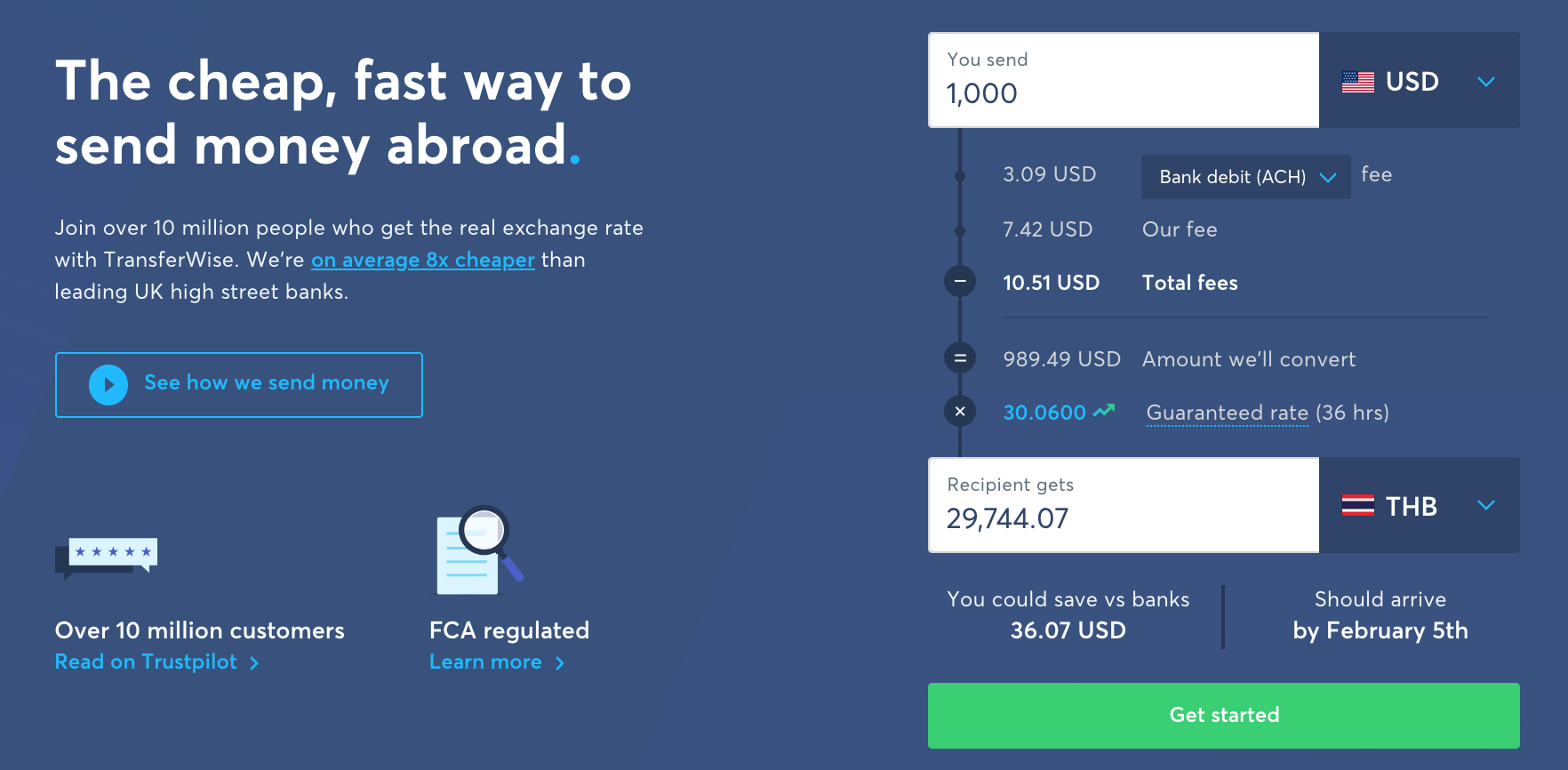The image is a blue rectangle oriented horizontally, featuring a detailed promotional message in white font. The main text reads: "The cheap, fast way to send money abroad. Join over 10 million people who get the real exchange rate with TransferWise. We are on average 8x cheaper than UK high-street banks," with "8x cheaper" distinctly highlighted in blue and underlined.

The image also features a prominent button labeled "See how we send money."

In addition, it highlights customer satisfaction with a note: "Over 10 million customers read on Trustpilot," with "read on Trustpilot" also in blue. The image assures users that the service is FCA regulated via a "Learn more" link in blue text.

The bottom section of the image contains a transactional illustration:
- A drop-down menu specifying the sending currency as USD ($1,000).
- The bank debit fee (ACH): $3.09 USD (indicated by a pull-down option).
- Total fees: $10.51 USD (broken down as $7.42 for TransferWise fees).
- Final converted amount: $989.49 USD.
- Guaranteed rate: $30.0600 within 36 hours.
- Recipient receives: ฿29,744.00 THB.
- Money saved versus banks: $36.07 USD.